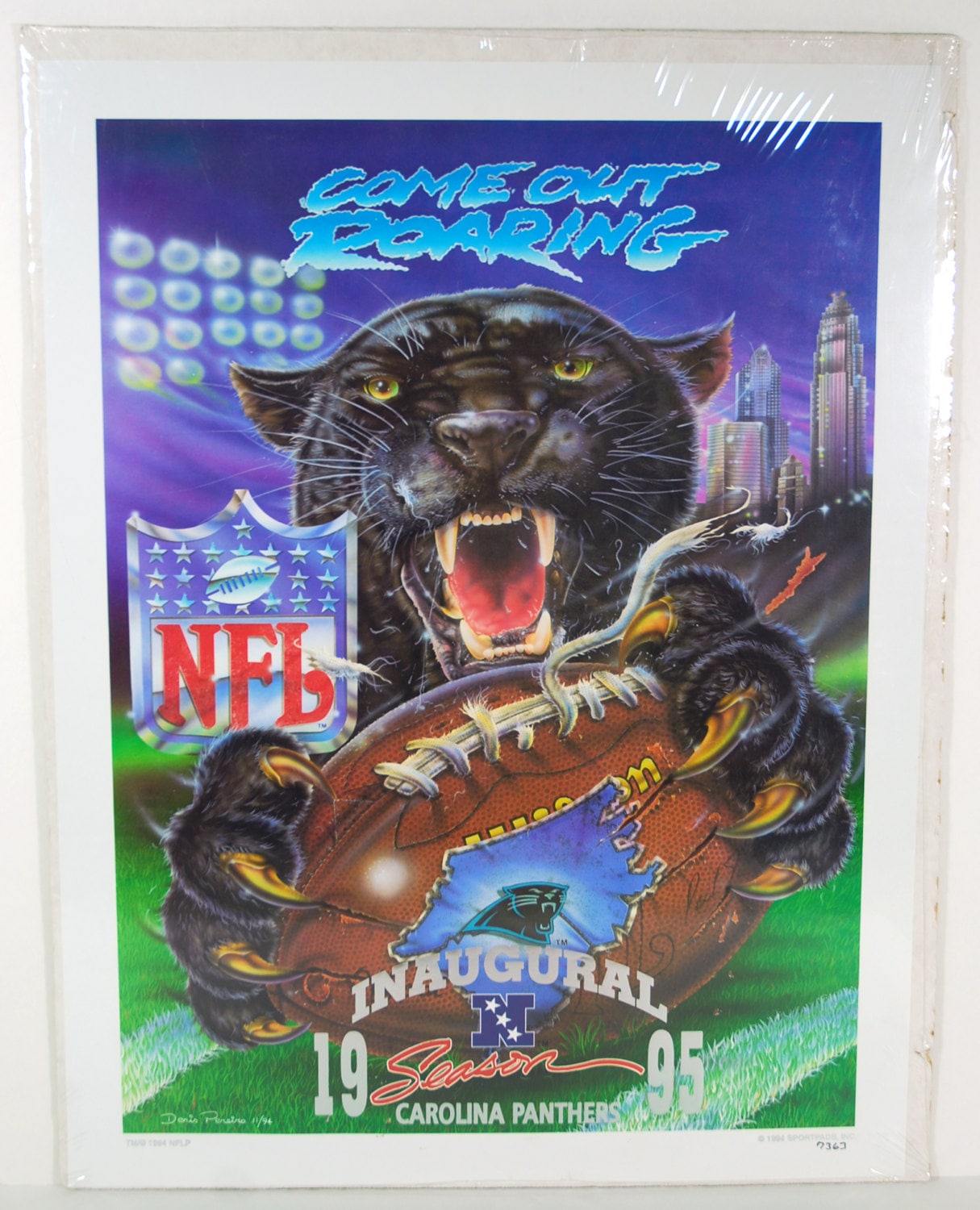The image is a detailed and collectible poster, reminiscent of something displayed in a stadium. The poster features a painted scene with a white border resembling a picture frame. Dominating the center is a giant black panther, the Carolina Panthers' mascot, holding a football that features the map of North Carolina. The backdrop showcases a skyline viewed in the evening, with buildings noticeably present on the right-hand side. At the top middle, in bold blue letters, the phrase "Come Out Roaring" is prominently displayed. On the left-hand side, the NFL logo is visible. At the bottom of the poster, in white letters, it reads "Inaugural 1995 Carolina Panthers Season," with the word "Season" highlighted in red.